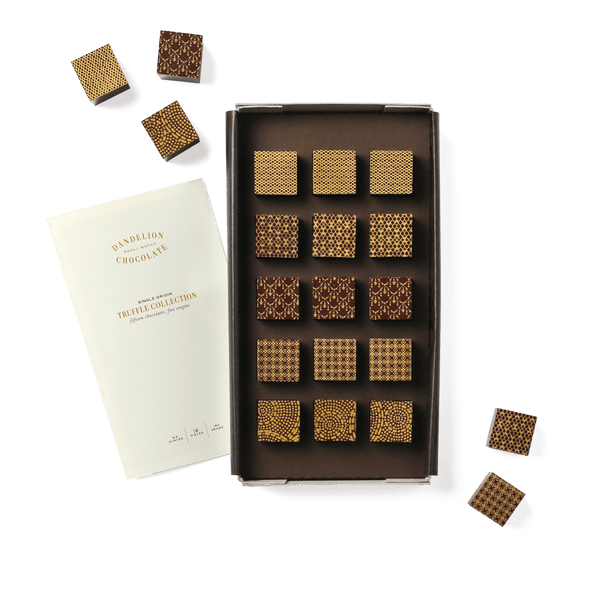The image features a luxurious box of Dandelion Chocolate Truffle Collection chocolates, set against an entirely white background reminiscent of a professional web page. The top of the dark brown box is off, revealing 15 truffles arranged neatly in five rows of three. Each square-shaped truffle sports a unique, symmetrical pattern—ranging from X's to waves to circles—etched in yellow details that complement the chocolates' rich brown tones. The patterns are slightly different but design-wise not significantly varied, lending an expensive and fancy appearance to the collection. Positioned next to the box on the left is a cream-colored pamphlet with golden-brown text, detailing the Dandelion Chocolate Truffle Collection. Additionally, several of the truffles are scattered around the box, showcasing their intricate designs outside their compartments, yet all matching those inside the box. Shadows accentuate the chocolates and box, adding depth to the pristine white backdrop.